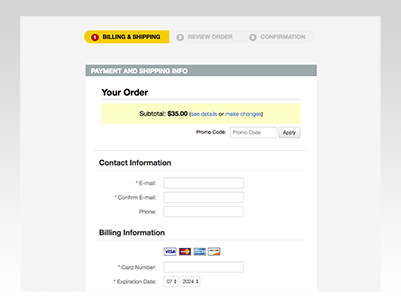The image depicts a screenshot of an online checkout page. The sections "Billing" and "Shipping" are highlighted in yellow, indicating the currently active part of the form, with a red background for emphasis. The stages "Review Order" and "Confirmation" are grayed out, suggesting these steps are not yet accessible. The form includes fields for payment and shipping information, displaying an order subtotal of $35 with options to "View details" or "Make changes." 

A section is available for applying a promo code, consisting of a box labeled "Promo code" and an "Apply" button. The contact information section contains fields for the user's email address, a confirmation box for re-entering the email, and a box for entering a phone number. 

Below this, the billing information section presents icons for Visa, MasterCard, American Express, and another unspecified payment method. An input box is available for entering the card number, followed by fields for the expiration date. The expiration date section features dropdown menus: one for the month with associated arrows for selection and another for the year, pre-filled with "2024" and navigation arrows.